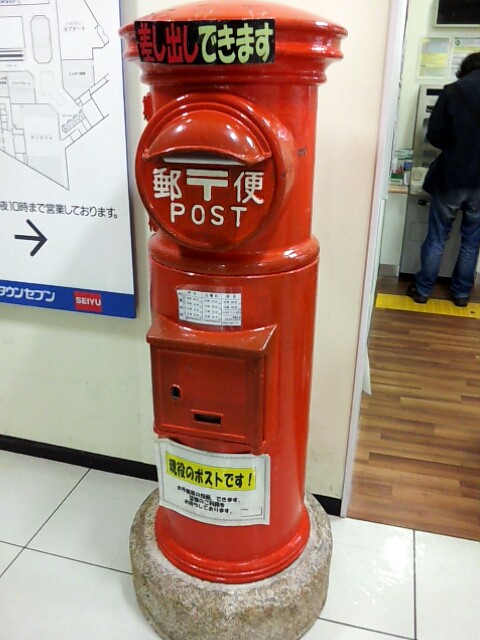The image depicts an indoor setting, possibly a post office, illuminated brightly by indoor lighting. The scene is largely divided between two types of flooring: white tile in the foreground and hardwood or laminate in the background. At the center of the image stands a shiny red mail post with Asian script along the top and bottom, suggesting it could be located in an Asian country. The mail post rests on a small circular stone base. Towards the top left of the image, a white sign, possibly a map, bears an arrow pointing to the right and the text "SEIYU," alongside additional Asian characters. In the top right, a man wearing blue jeans and a black coat stands on a yellow section of the floor, interacting with a machine, perhaps part of the mailing process. The image is rich in color, featuring shades of white, black, off-white, blue, red, and yellow.